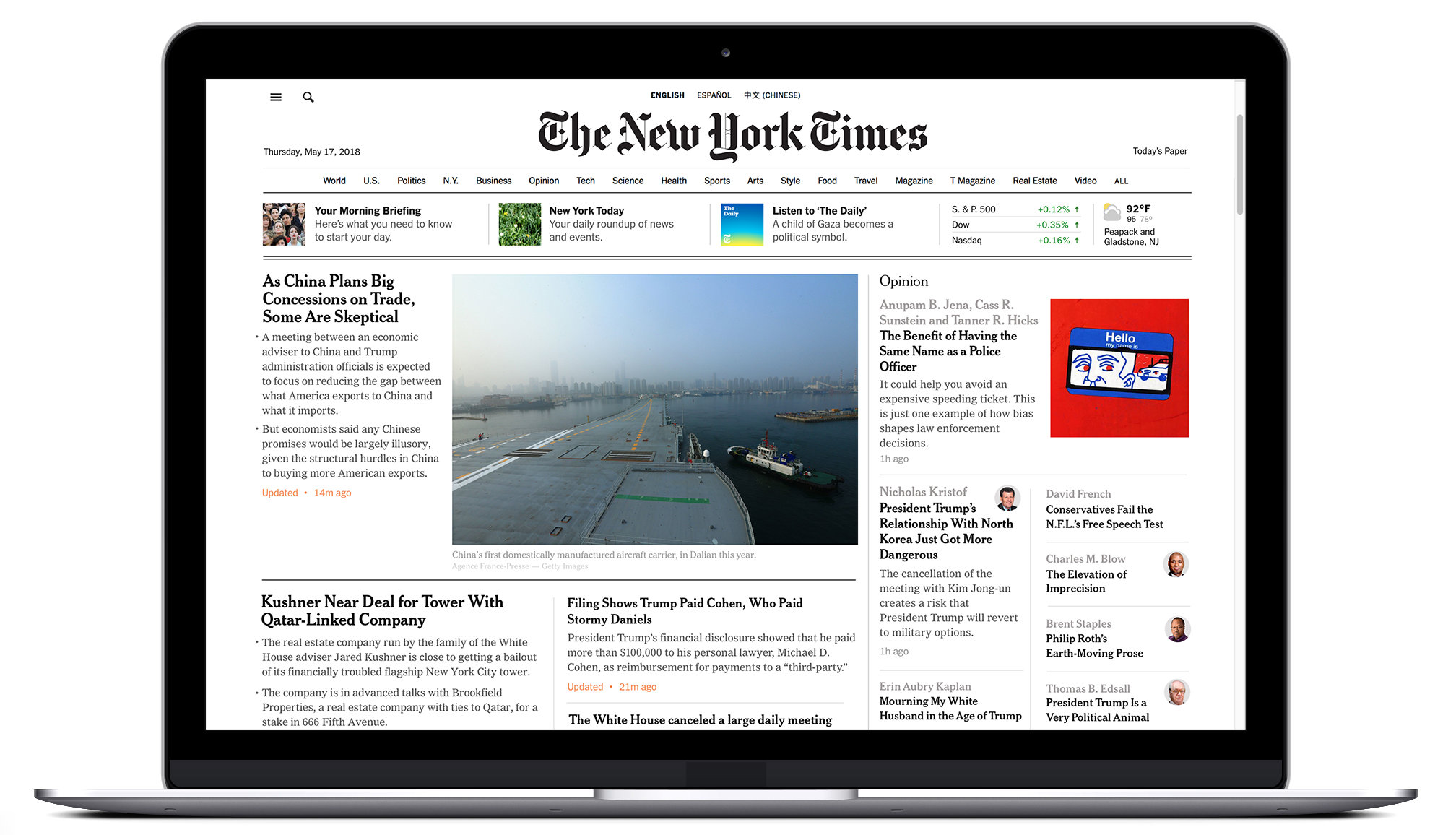The image depicts a laptop computer screen displaying a page from the New York Times website. At the top of the screen are a hamburger menu icon and a search icon, flanking the date, Thursday, May 17, 2018. To the right of the date is a link labeled "Today's Paper." 

The page is organized into various sections. From left to right, the first section appears to be "The Morning Briefing," followed by "New York Today," and "Listen to The Daily." Financial updates for the Dow and NASDAQ are shown alongside the temperature, which is indicated as 92 degrees Fahrenheit. Below these sections are several news articles.

In the primary news section, there is an image of a waterway with what seems to be an aircraft carrier, possibly being maneuvered by towboats. The headline above this image reads "As China Plans Big Concessions on Trade, Some Are Skeptical." 

Beneath this main article is another headline: "Kushner New Deal for Tower With Qatar-Linked Company." To the right of this, another headline reads: "Filing Shows Trump Paid Cohen, Who Paid Stormy Daniels."

Lower on the page, another headline notes: "White House Canceled a Large Daily Meeting." To the right are various opinion pieces, including titles like "The Benefit of Having the Same Name as a Policy Offer," "President Trump's Relationship With North Korea Just Got More Dangerous," "Mourning My White Husband in the Age of Trump," "Conservatives Fail the NFL Free Speech Test," and "The Evidence of the Evaluation of [incomplete]."

This detailed webpage structure gives an overview of the top stories and sections from the New York Times on that particular day.